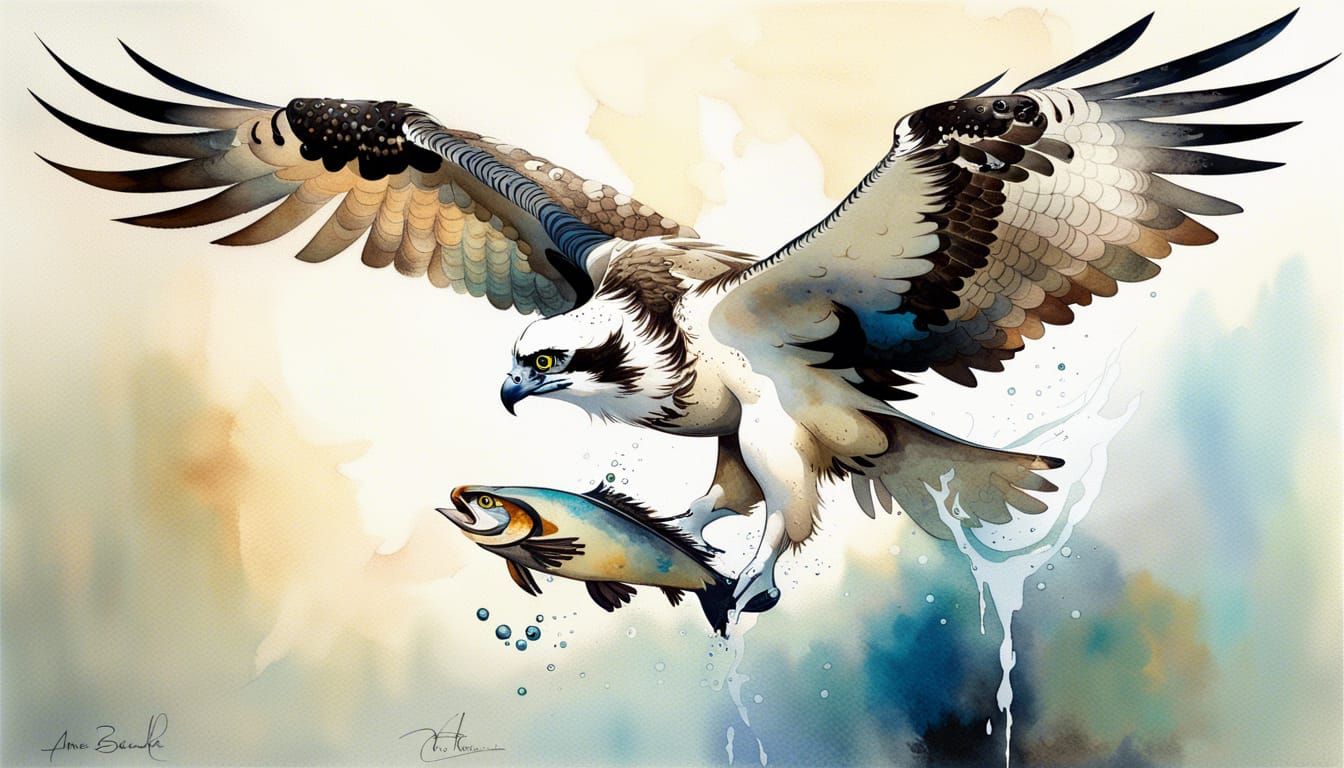This is a detailed, artistic watercolor painting of an eagle with a fish tightly gripped in its talons. Both the eagle and the fish face towards the left side, and the scene captures the moment right after the eagle has snatched the fish from the water, evidenced by droplets cascading off the bird. The eagle is depicted with a white feathered head and has wings that are predominantly yellow with black accents, resembling those of an osprey. The background of the painting exhibits a blend of warm sunny yellows and oranges interspersed with darker blues and greens, creating a dynamic and colorful backdrop. The fish in the eagle’s grip displays varying shades of blue, from dark to light, adding to the visual diversity. Additionally, the eagle’s body has brown and beige feathers, showcasing the artist’s keen attention to detail. This image is signed twice in cursive, once in the bottom left corner and once just left of center at the bottom, indicating the artist's authentication of their work. The overall atmosphere of the painting is focused and intense, highlighting the eagle’s concentration and skill as a hunter.